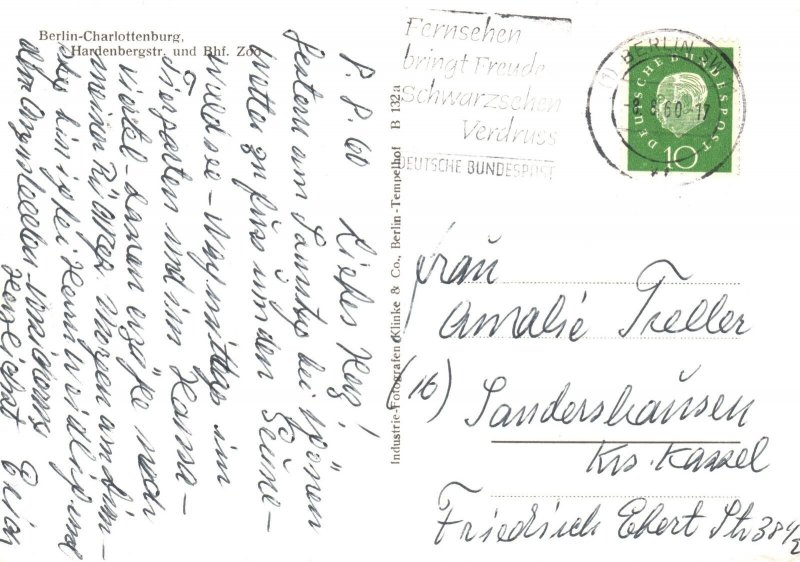This rectangular image, oriented with its long side stretching from left to right, depicts a vintage postcard that has been written, sent, and postmarked. The postage stamp, positioned in the upper right-hand corner, is green and features the profile of a person's face along with the denomination "10." A postal marking overlays the stamp, reading "Berlin SW." Adjacent to this, another postmark to the left states "Verschenringfrühde Schwartzenschenverduris," suggesting German origin.

Continuing leftward, additional postmarks indicate "Berlin, Charlottenburg, Hartenberg" and "UNDBHF.ZOO." Below these markings, unreadable text written vertically occupies the entire left-hand side, contrasting with the horizontal orientation of the image. Directly under the postage stamp on the right side is the address section, also inscribed in German and beyond the writer's comprehension. This detailed scene evokes a sense of historical communication, providing glimpses into the postal practices and geography of early 20th-century Berlin.